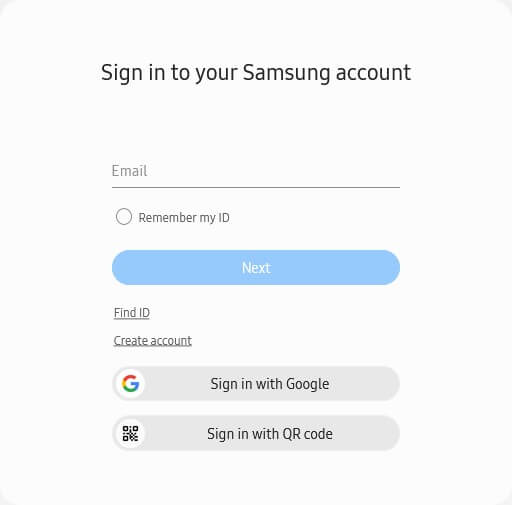The image features a screenshot of the Samsung account sign-in page. The background is predominantly off-white, creating a clean and simple aesthetic. At the center, text is center-justified, displaying "Sign in to your Samsung account" in a medium gray, regular font.

Below the heading, there is a blank field labeled "Email" where users can type in their email addresses. Adjacent to this field, an option to remember the user’s ID is present, ensuring convenience for future logins from the same device. 

A prominently displayed, large, light blue button with rounded edges and the word "Next" in white is provided for users to proceed with their sign-in. Underneath this Next button, there are links for retrieving a forgotten ID or creating a new account, each accompanied by their respective clickable buttons.

Additionally, alternative sign-in options are available at the bottom. Users can sign in with their Google accounts, signified by the Google logo and a button, or utilize a QR code sign-in method, indicated by a QR code symbol. This facilitates multiple ways to access the account, highlighting Samsung's inclusivity in accommodating different user preferences.